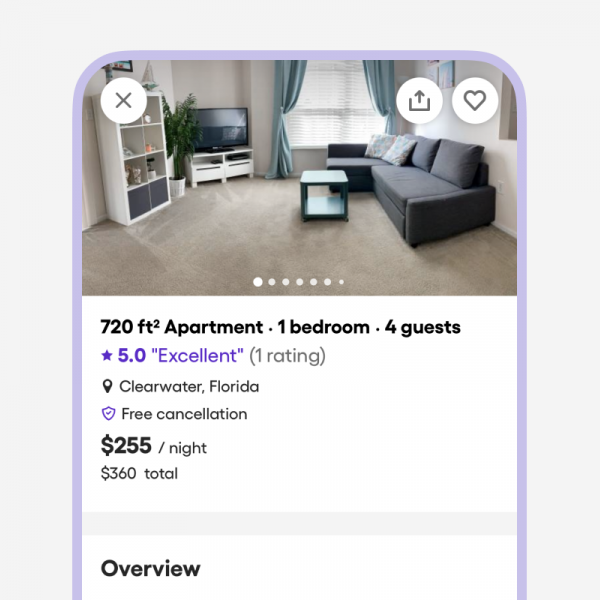This image is a detailed screenshot of an Airbnb listing displayed against a light gray background with a rounded light purple outline, mimicking the shape of a mobile device screen. Dominating the top section of the listing is an inviting image of a chic living room. The image features three interactive buttons positioned in white circles at the top-left corner: an 'X' for closing, an upload button, and a heart outline symbolizing 'favorites.'

Below the image, seven small dots indicate the presence of additional photos available for swiping. The listing information is presented on a crisp white background, starting with the property details: "720 square feet apartment, one bedroom, accommodates four guests," in bold black text. Following this, a review rating is highlighted in blue with a star icon, showing "5.0" alongside the word "excellent" in quotation marks, and a note "(1 review)" in gray.

Additional icons beneath provide further insights, including a map icon revealing the location as Clearwater, Florida, and a note about the "free cancellation" policy. The pricing information is clearly stated: "$255 per night" and "$360 total."